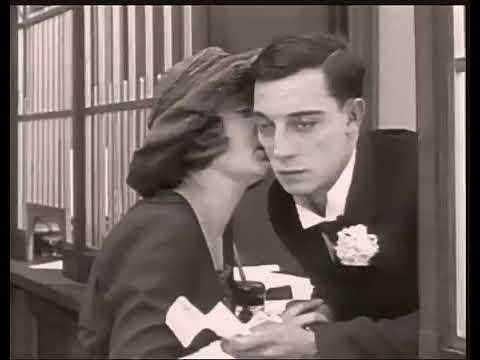In this black-and-white image reminiscent of a still from an old-fashioned movie, a man and a woman are the central figures, framed by a thin black border. The man, visible from the chest up, is dressed in a long-sleeved black coat with a white button-up shirt and a black bow tie, adorned with a white flower on his left lapel. His slicked-back hair is parted to the side. In his left hand, he holds a wrinkled piece of paper, possibly a receipt.

The woman, also visible from the chest up, leans in close to the man, whispering in his ear, her face obscured by his. She wears a dark-colored top and a loose, cloth-looking hat, with shoulder-length curls peeking out. The setting suggests a bank teller's window or some kind of transaction counter, implied by the wooden panels and bars visible on the left side of the image. The scene conveys an air of secrecy and intimacy between the two characters, enhanced by the grayscale tones and vintage aesthetic of the photograph.